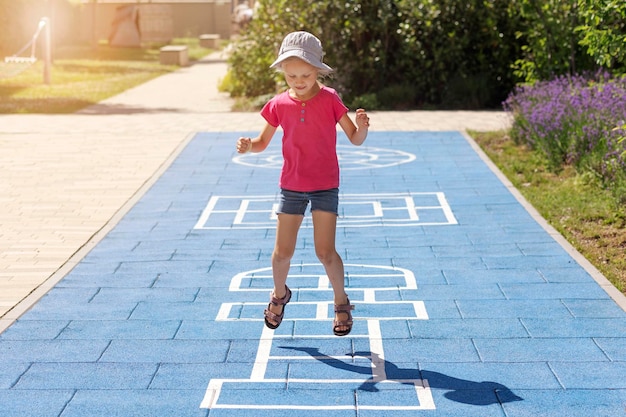The image captures a lively scene of a little girl appearing to play hopscotch on a blue-tiled walkway, adorned with white chalk or paint markings resembling a hopscotch board, though it lacks numbers. She is mid-jump, both feet in the air, looking down at her feet with an expression of joy. The girl, who is likely around five or six years old, has blonde hair and wears a pink polo shirt, jean shorts, sandals, and a hat. To her left, there is a grey sidewalk that extends away from her, while to her right, a patch of grass adorned with purple flowers is visible. Further in the background, to the upper left, there is a lawn area with benches and possibly statues, surrounded by shrubbery and more greenery. The overall setting hints at a park-like area, adding to the cheerful atmosphere of the scene.